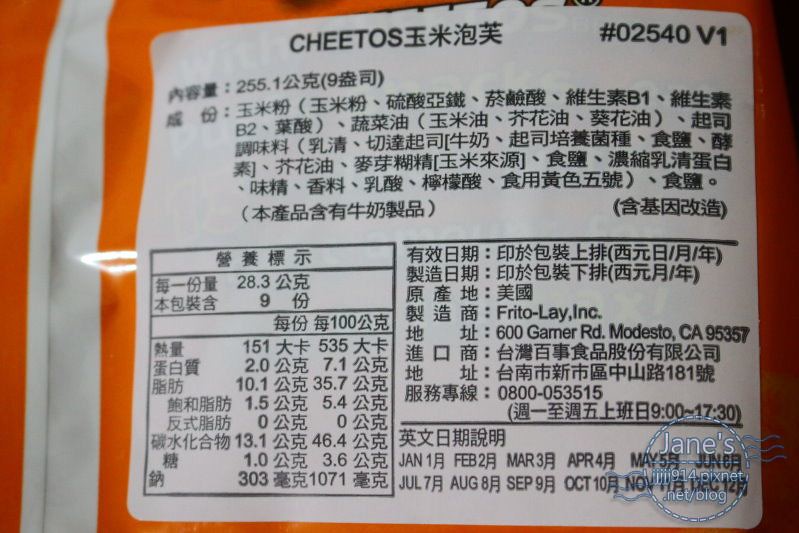This image features a white product label with black lettering, adhered to an orange and white plastic package. The package appears to be a bag of Cheetos. The top of the label prominently displays the word "Cheetos" in black ink. The text on the label is primarily in Chinese, and includes both nutrition and ingredient information, as well as various numbers such as 28.3, 9, 151, 535, 2.0, 7.1, 10.1, 37.5, 1.5, 5.4, 0, 0, 13.1, 46.4, 1.0, 3.6, 303, and 1071.

The label also includes the product's manufacturing information from Frito-Lay Incorporated, located at 600 Garner Road, Modesto, California. Additionally, there are several expiration dates listed towards the bottom right corner of the label, from January through December 2015. The label is placed on the orange-colored bag that features a white stripe running vertically from the top to the bottom along the left side. An icon or inscription marked "Jane's" in blue is enclosed within a circle at the lower right of the label.